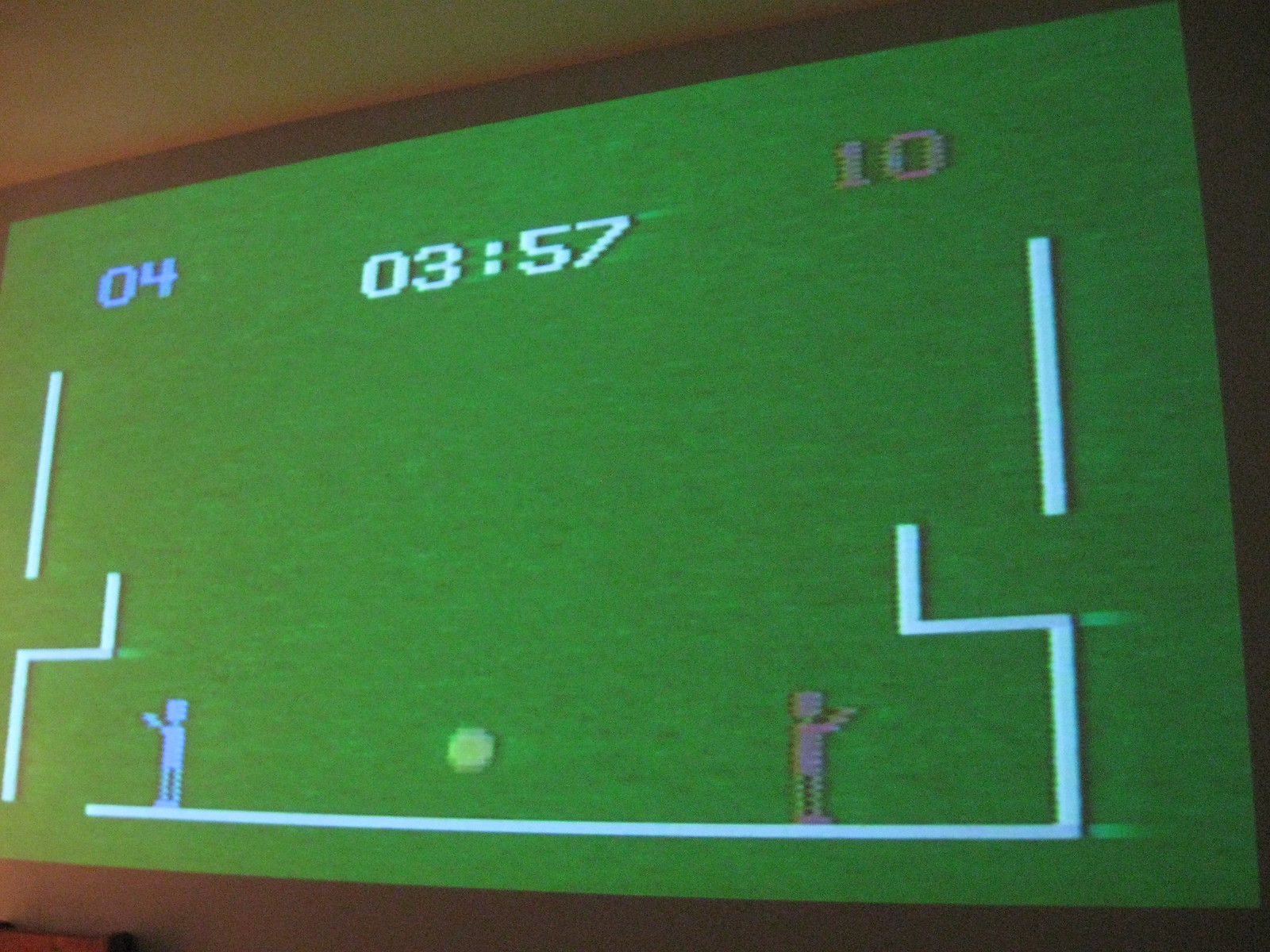The image showcases a screenshot of a retro-style video game displayed on an expansive green screen, which appears to be the primary source of illumination in an otherwise dark background. The screen prominently features a score display at the top with the numbers "04" in light blue on the left and "10" in dark gray on the right. A timer beneath the scores indicates that there are "03:57" minutes remaining in the gameplay.

In the foreground, two stick figures stand on a zigzagging white line at the bottom of the screen. The figure on the left is blue, while the one on the right is red, both pointing in opposite directions. Between them is a yellow ball, which seems to play a central role in the game. The green screen is punctuated with various white lines: two vertical ones at the top corners extending downward, and another squiggly line to the left that rises slightly before angling to the right.

The scene evokes a sense of nostalgia with its primitive graphics, comprising blocky, maze-like segments and stick figures. It is uncertain what the exact objective of the game is, but the red player appears to be leading, according to the score.